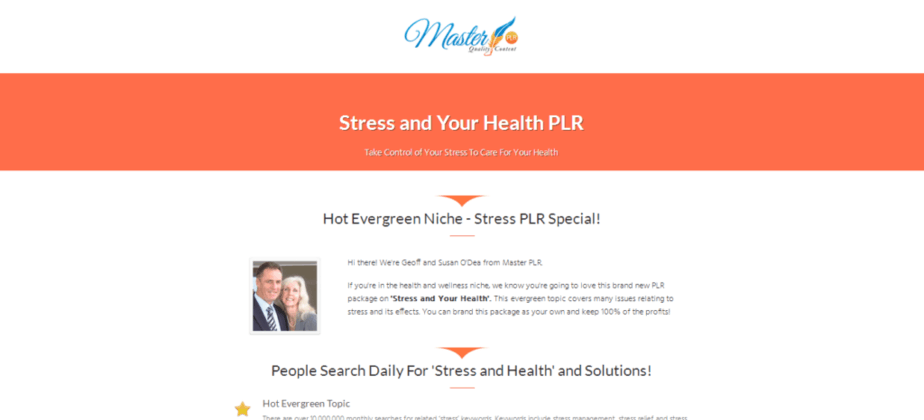Screenshot of a desktop website showcasing a layered vertical layout. At the top, a logo features the word "Master" in blue, accompanied by an intricate design incorporating orange and blue elements and a smaller, unreadable text. Beneath the logo section, an orange background with bold white text reads, "Stress and Your Health PLR: Take Control of Your Stress to Care for Your Health."

Following this, a white background displays black text proclaiming, "Hot Evergreen Niche: Stress PLR Special." On the left side of this section, there is an image of a man and woman who appear to be Jeff and Susan Odea, with a caption introducing them and stating, "Hi there, we're Jeff and Susan Odea. If you're in the health and wellness niche, we know you're going to love this brand new PLR package on stress and your health." 

Below their introduction, a final line emphasizes the relevance of the content: "People search daily for stress and health solutions."